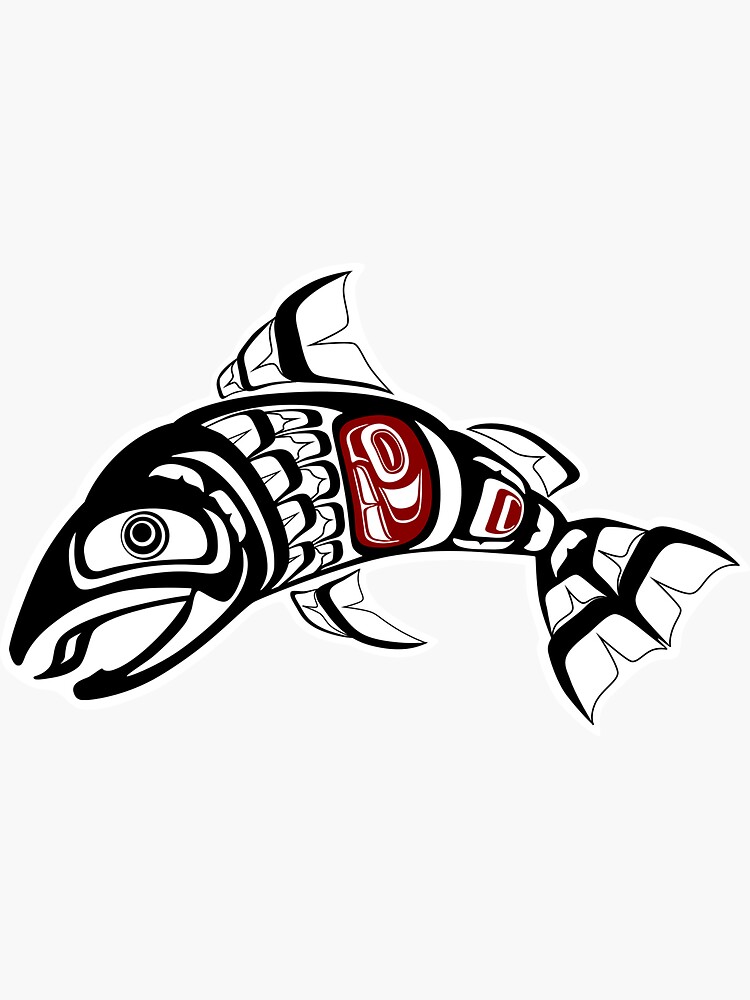This image features a meticulously drawn but non-realistic, fantasy-themed fish set against a gray background. The fish, which appears in black and white with selective red accents, exudes a whimsical yet deliberate design that could serve as a logo, an advertisement for a sushi restaurant, or even a potential tattoo sketch. The fish is depicted in a dynamic pose, curving as if leaping out of the water, and has no teeth. Its mouth is open, it showcases a black eye, and the body is adorned with black and white scales. Notably, the stomach area and a portion of the tail fin exhibit red and white decorations, adding a vivid contrast to the monochrome theme. The exterior features outlined fins and a discernible tongue, while the center appears to include some letters, potentially a C or a D, suggesting an artistic or branded element. Overall, the image captures an artistic rendering of a fish with intricate details and an imaginative flair.